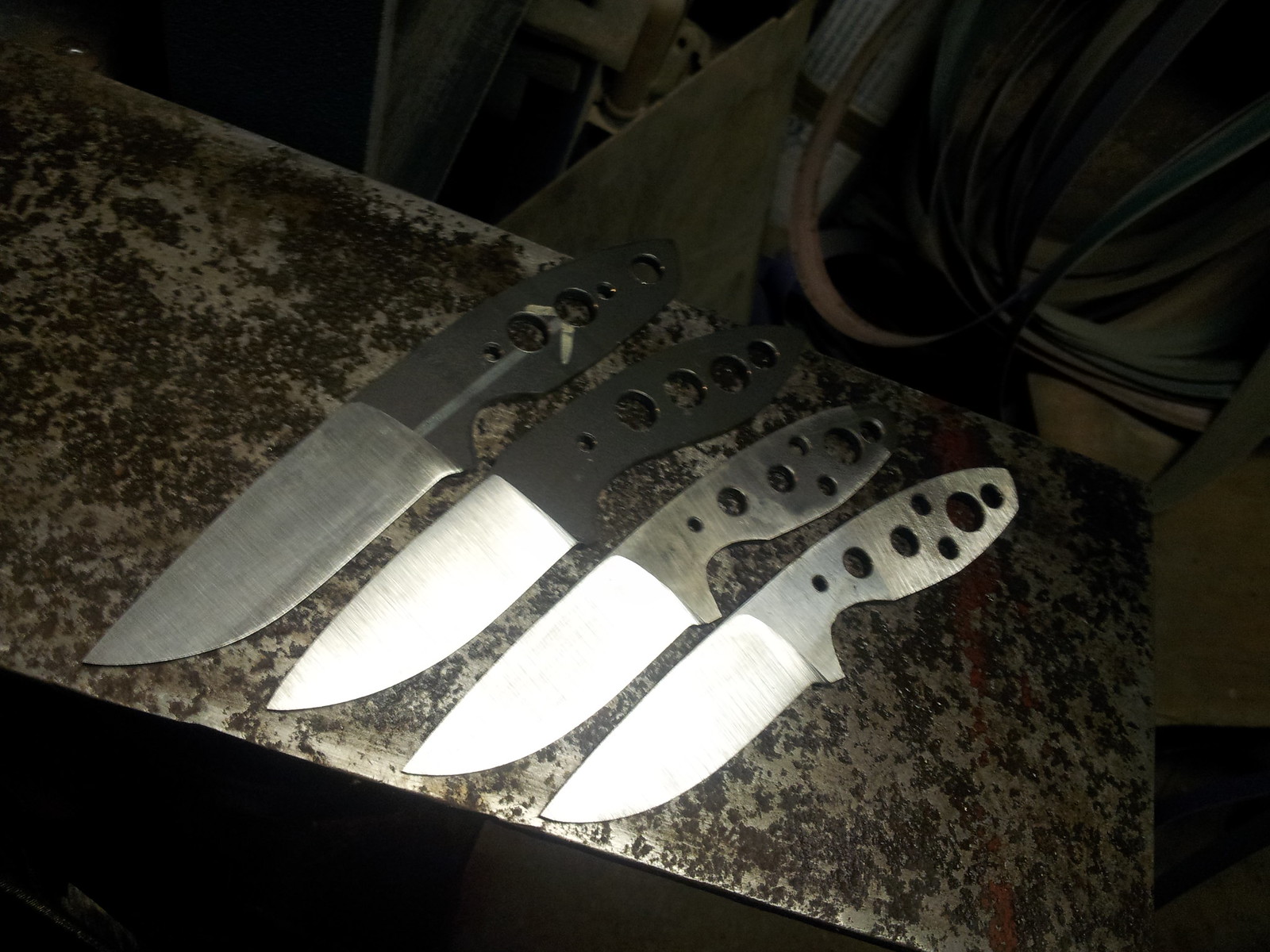This photograph depicts a dimly lit scene featuring four hunting knives neatly laid out on a rusted metal shelf or sheet situated in the interior of what appears to be a truck or van, possibly inside the central console area between the seats. The grayish metal surface displays splotches of darker gray, suggesting significant wear and age. The knives are aligned from left to right, decreasing in size.

The largest knife on the far left is entirely metallic with a visible blade, whereas the remaining three knives, progressively smaller towards the right, have blades that seem to be covered with white sheaths. Among these, the two leftmost knives (besides the largest one) have black-finished handles, in contrast to the rightmost two knives which have matte stainless steel handles. All handles are perforated with variously sized holes, contributing to their intricate, patterned design.

In the backdrop, elements like tubing or hoses suggest the setting might be a garage or workshop. Also visible is a granite slab with brown, red, and gray hues, adding to the rustic atmosphere. Additionally, bands that appear to be sanding belts, possibly intended for a loop sander, are seen, further reinforcing the industrial context.